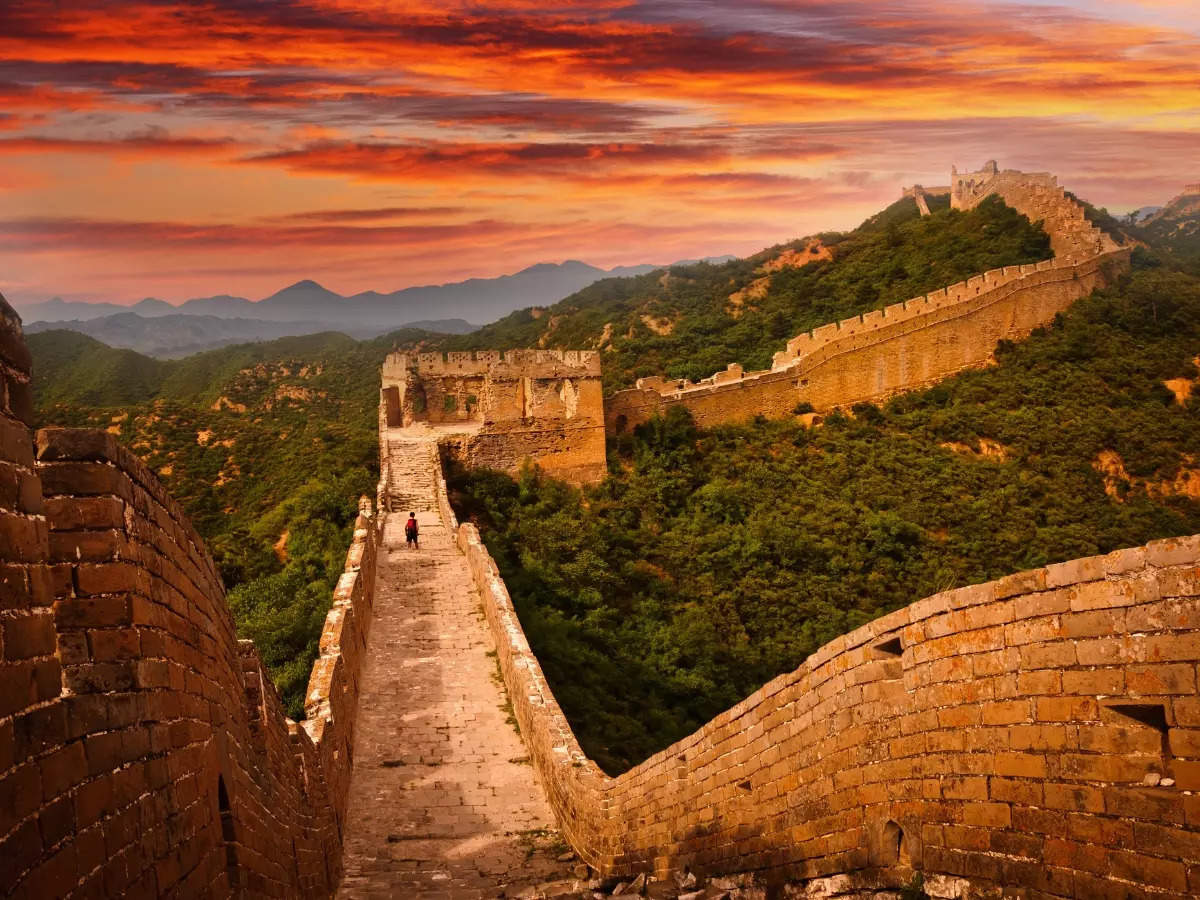This photograph encapsulates a breathtaking view of the Great Wall of China, taken from a high vantage point that looks down onto the ancient stone and brick structure. The wall starts in the center of the image, snaking its way to the upper right, surrounded by lush green trees on all sides, which make up a vast, verdant valley. In the middle of this historic pathway, there is a small figure wearing a red shirt and dark pants, likely a young boy, who stands alone, adding a sense of scale and solitude to the scene. The wall is punctuated with little holes, possibly meant for defense purposes, through which guards may have once stood. The backdrop features a stunning, unique sunset sky painted with waves of reds, purples, yellows, and lilacs, casting a colorful glow over distant mountains, making it a picturesque landscape.